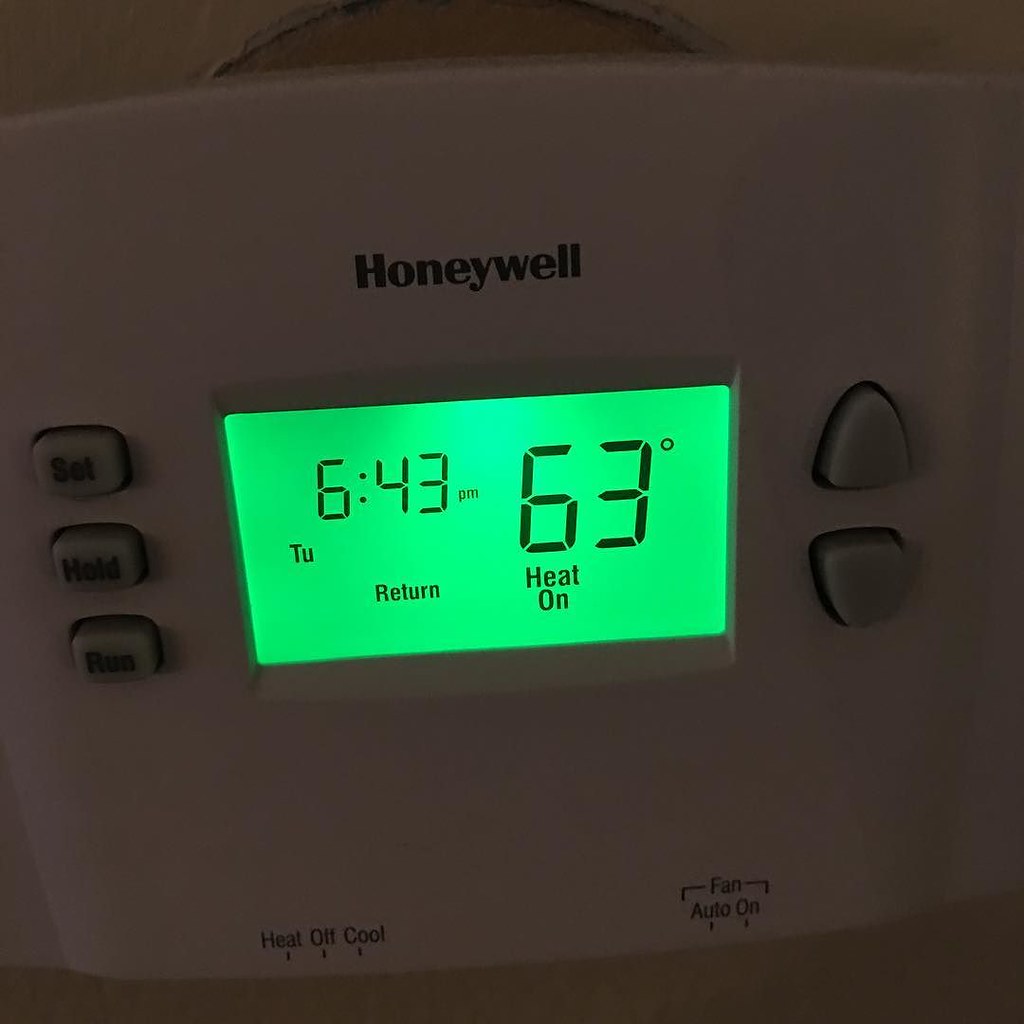This detailed caption describes a highly zoomed-in image of a digital thermostat set against a wall inside a home. The wall appears to be of a darker hue compared to the thermostat—possibly off-white to gray. The white plastic thermostat prominently features the brand name "Honeywell" inscribed in black text at the top. 

On the left side of the device, there are three vertically arranged gray, rubbery-textured pushbuttons labeled "Set," "Hold," and "Run." The right side houses two gray, arrow-shaped buttons for adjusting settings, with one button pointing up and the other pointing down.

At the bottom left section, options for "Heat," "Off," and "Cool" are listed vertically, each with corresponding lines to indicate switch positions. To the bottom right, the "Fan" settings offer "Auto" or "On" options.

The digital screen is brightly lit in green, displaying essential information: the current time "6:43 PM," the day "TU" (indicating Tuesday), the status "Return," and the temperature setting "63 degrees" with "heat on."